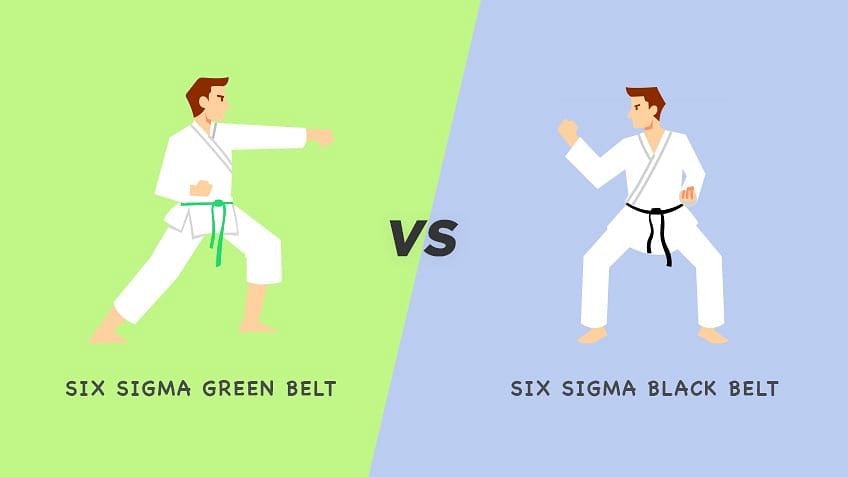The image is a cartoon drawing depicting two Caucasian men in martial arts stances, both wearing karate uniforms. The left side of the image features a green background where a man with short brown hair, dressed in a white karate outfit and a green belt, is positioned with his left arm extended forward and his right arm pulled back into a fist. Below him, black text reads “Six Sigma Green Belt.” The right side has a lavender background and shows another man, similarly dressed but with a black belt, in a defensive stance with his arm bent and fist out. Below him, it also says “Six Sigma Black Belt” in black text. The two individuals are facing each other, suggesting a comparison or confrontation.